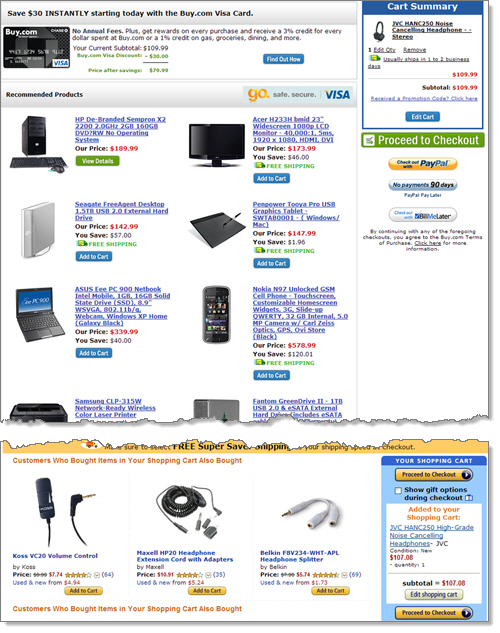This is a detailed screenshot of a product page from Buy.com, featuring a two-column layout. At the top left, a prominent gray bar stretches across the page with the message: "Save $30 instantly starting today with the Buy.com Visa Card." Next to this message, there's an image of the sleek Black Buy.com Credit Card Visa. 

To the right of this announcement, the text highlights the card’s benefits: "No annual fees, plus get rewards on every purchase and receive 3% credit for every dollar spent at Buy.com, or 1% on gas, groceries, dining, and more."

On the right side of the screenshot, there's a sidebar. At the top of this sidebar, a blue header marked "Cart Summary" in white stands out. Directly below, a picture of a pair of headphones is displayed. The total cost is shown in bold red text as $109.99, followed by a red subtotal of $109.99. 

Beneath this, there's a blue link reading, "Received a Promotion Code? Click here." Below this link, a blue "Edit Cart" button is available, followed by a "Proceed to Checkout" button, which includes various payment options icons.

On the left side of the page, in the main content area labeled "Product Page," there are two columns showcasing different products. The user is prompted to click "Electronics" to explore that category further.